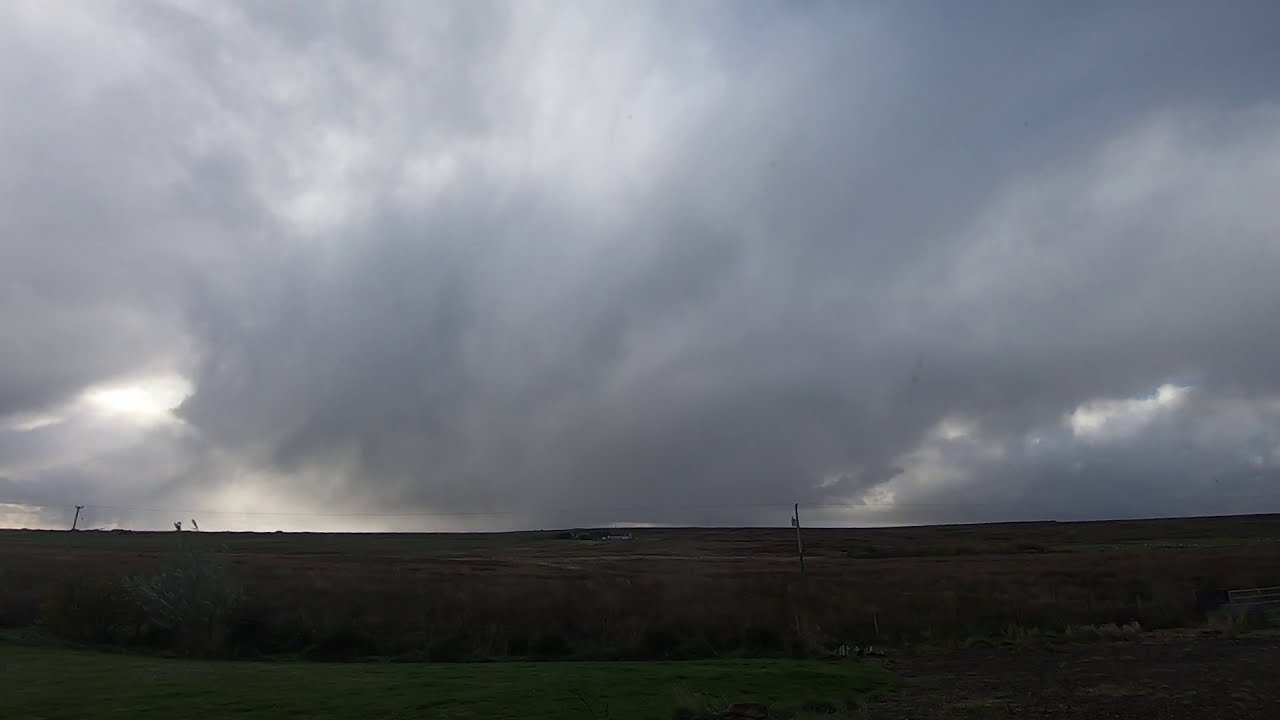This photograph captures a dramatic outdoor landscape dominated by a vast, cloudy sky. Thick, heavy storm clouds in shades of gray, dark blue, and black mix with patches of white, covering two-thirds of the image. In the lower left corner, a sliver of light breaks through the sky. The bottom third of the photo features an expansive, mostly weed-covered grassy field, gently curving at the edges. A dirt patch is visible to the lower right. Scattered far across the horizon are small, barely discernible electrical utility poles or telephone poles, adding a sense of depth and distance to the scene. Overall, the cloud-filled sky is clearly the focal point, with its dynamic and shifting formations, hinting at the turbulent weather.